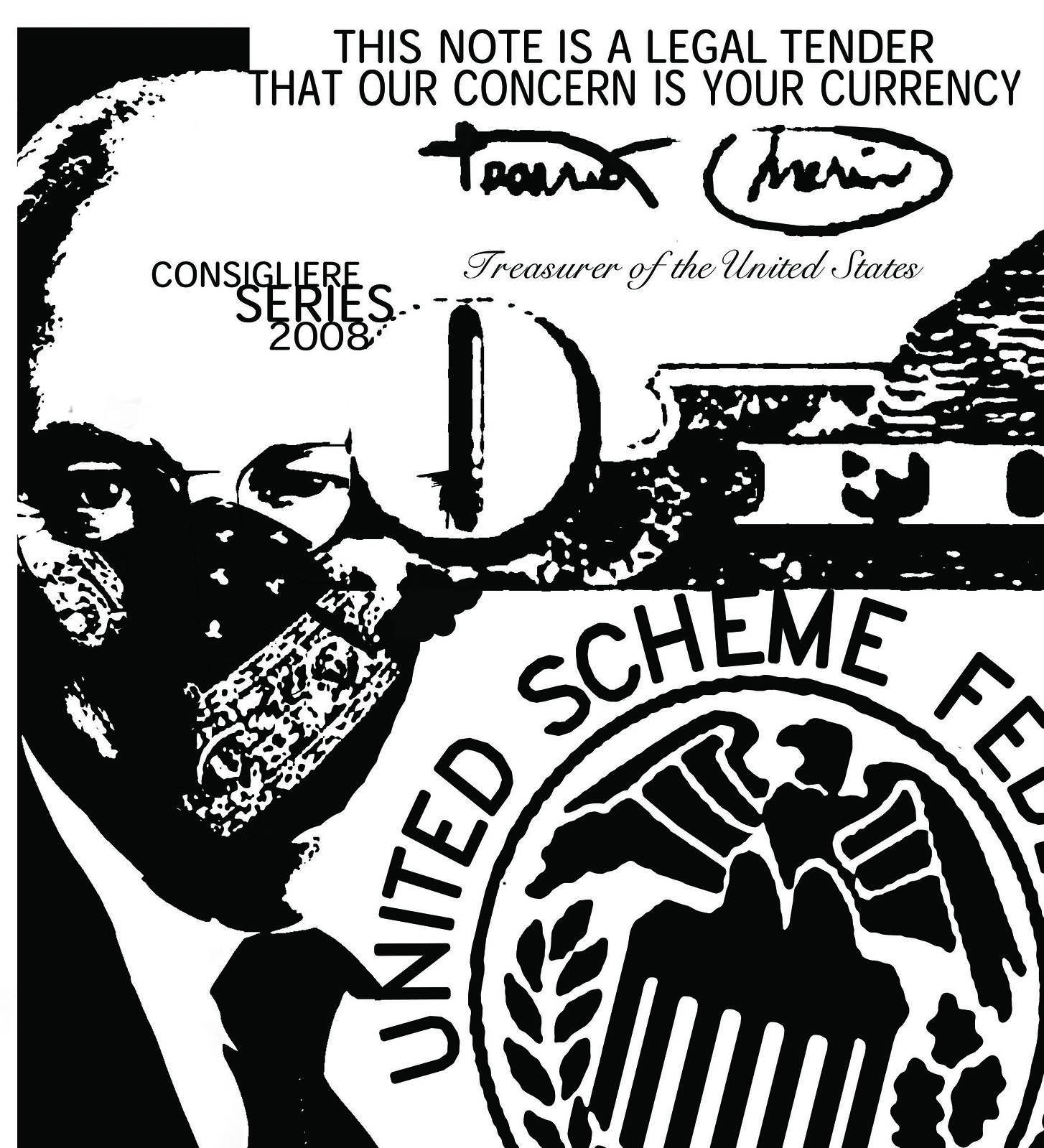This black-and-white image features a series of striking elements. At the top, bold text reads, "This note is legal tender that our concern is your currency," pointing to a potential political statement. Beneath this, the phrase "Consigliere Series 2008" is accompanied by two illegible signatures and the title "Treasurer of the United States" in cursive. The left side of the image displays a partial view of a man's head and upper body; his eyes are visible above a mask or bandana covering his mouth, and he wears a suit with a tie. To the right, there is a circular emblem featuring a bald eagle, reminiscent of the American Eagle found on coins, encircled by the words "United Scheme." The eagle seems to be perched on a structure, surrounded by olive leaves and other foliage, adding to the intricate, edited design of the artwork.